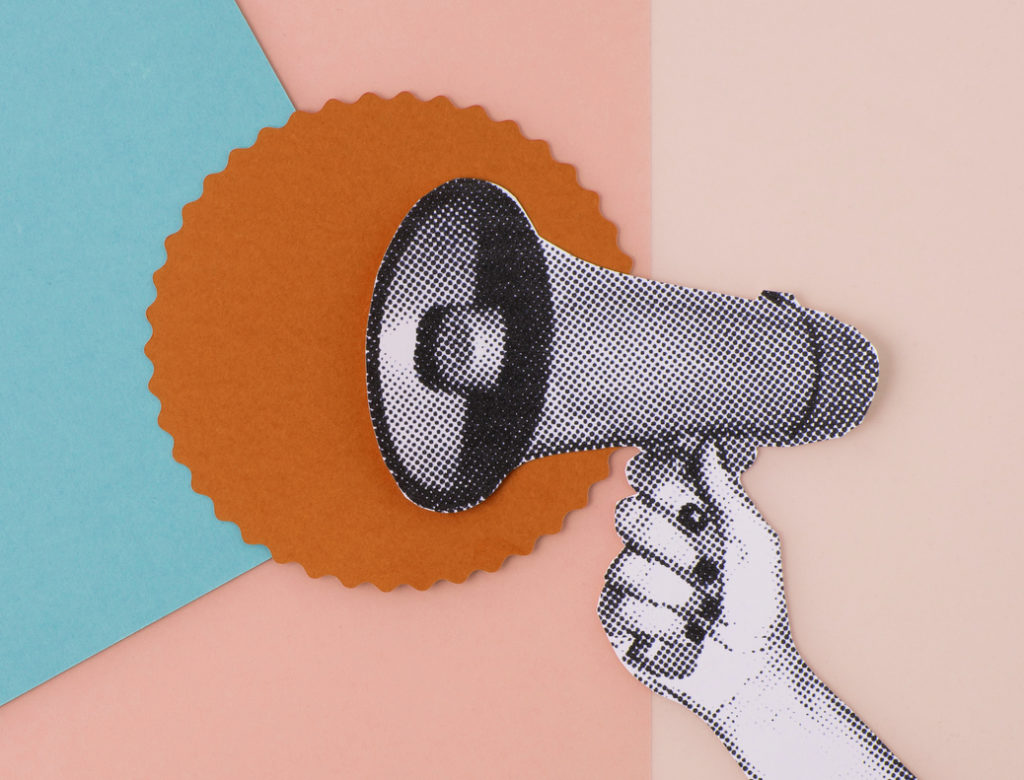The image depicts a meticulously crafted paper collage, showcasing multiple layers and intricate details. At the base of the collage, there is a sheet of light pink paper visible primarily on the right side. Layered over this is a darker salmon pink paper, covering the midsection. Diagonally placed on top is a turquoise paper, extending across the left side. Central to the artwork lies a circular cutout in orangish-brown, featuring a ridged, scalloped border, reminiscent of a felt texture. In the foreground, a black-and-white pixelated megaphone, rendered with small detailed boxes, is held aloft by a hand with painted fingernails, suggesting it may belong to a woman. The megaphone, appearing silver and black, is directed toward the right side, giving the composition a dynamic element.